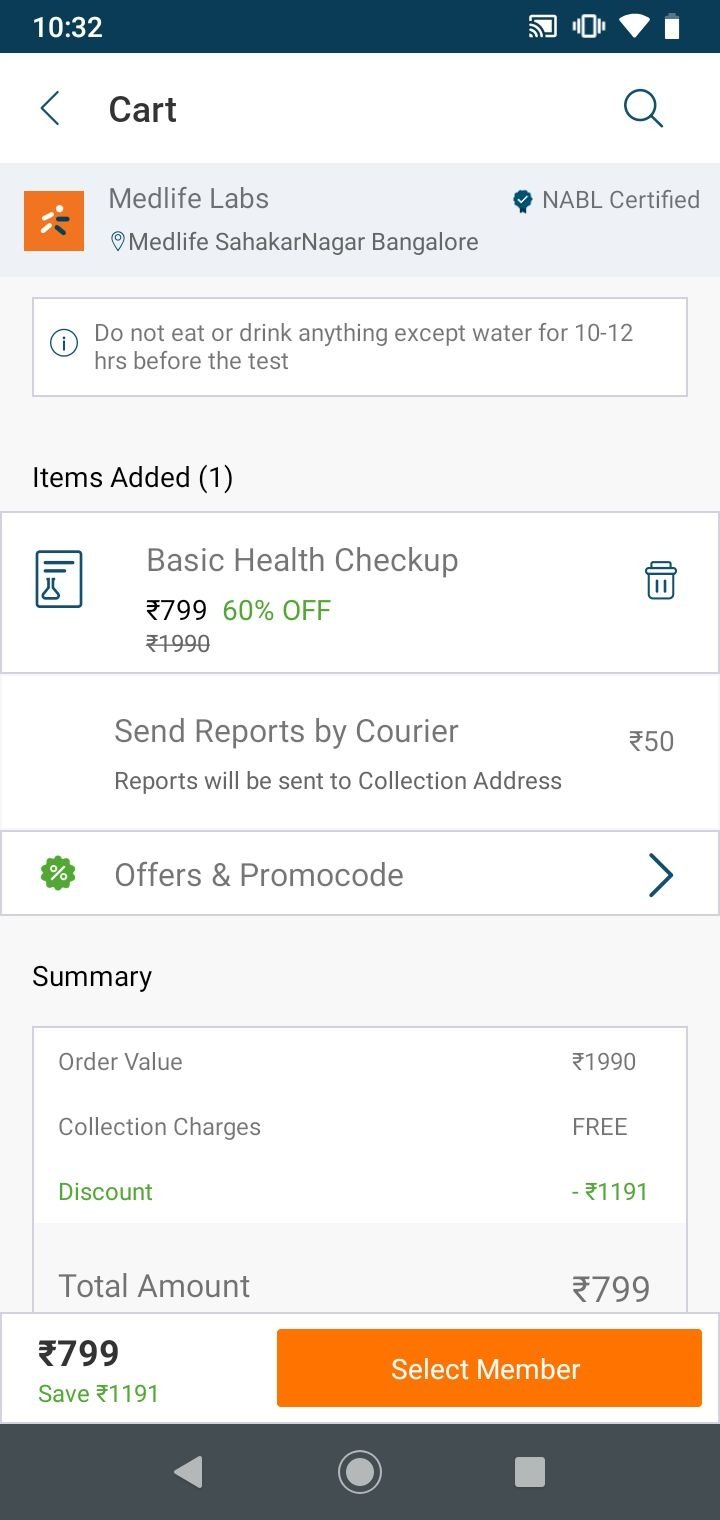The screenshot displays a mobile phone screen taken at 10:32. At the top of the image, there is a status bar featuring several elements: a time indicator, signal strength icon (represented by three curved lines within a rectangle), Wi-Fi symbol, phone battery level showing full charge, and various service icons. 

Below the status bar, within a white rectangular toolbar, the word "Cart" is visible in black font, accompanied by a back arrow on the left and a magnifying glass icon on the right.

The main content area showcases an orange square with a dynamic stick figure icon indicating movement. Beside this graphic, "Medlife Labs" is written in bold letters, and below it, the location "Medlife Shaharqa Nagar Bangalore" is mentioned. Adjacent to this, a verified check mark is shown with the certification "NABL certified," emphasizing the lab's accreditation.

A cautionary notice follows, advising: "Do not eat or drink anything except water for 10 to 12 hours before this test." Further down, a section labeled "Items added" lists a "Basic Health Checkup" with a striking "60% off" in green font. A trash can icon next to this entry allows for removal of the item.

Subsequently, an option is displayed: "Send reports by courier," with a note that reports will be sent to the collection address for an additional charge of 50. Below the items section, there's a segment for "Offers and promo code," featuring a flower-shaped icon with a percentage sign.

Finally, the cost breakdown is presented with fields for "Order value," "Collection charges," "Discount," and "Total," summarizing the transaction details.